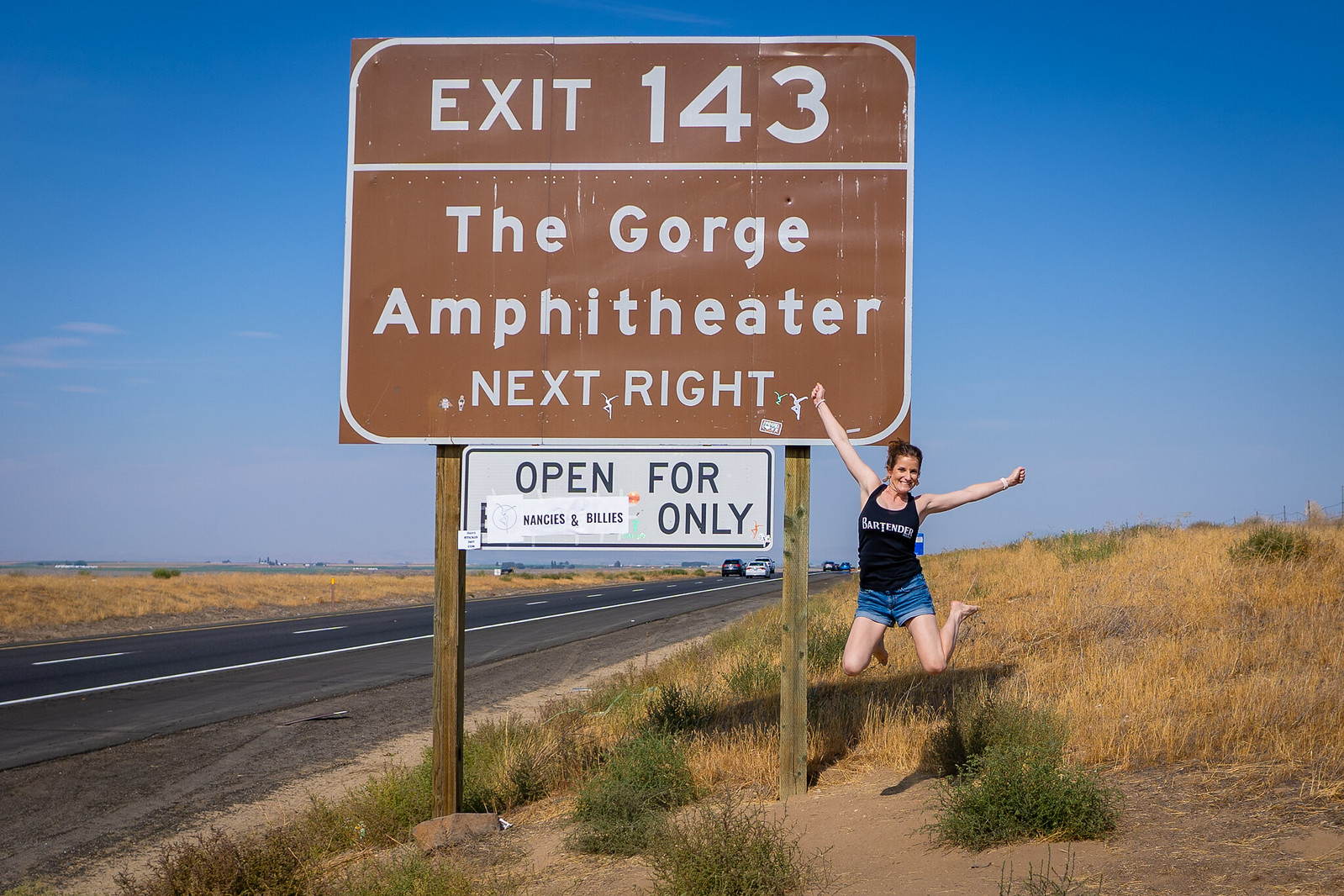This photo captures an exuberant moment along a stretch of highway near Exit 143 for the Gorge Amphitheatre. The sky is a clear, vibrant blue with very few clouds, highlighting a bright, sunny day. The landscape is dominated by brown grass interspersed with patches of green. Prominently displayed is a brown highway sign with white lettering that says "Gorge Amphitheatre Next Right." Below it, an attached white sign with dark font reads "Open for Nancy's and Billy's Only," although part of this message appears to be obscured. 

In the foreground, a woman is caught mid-jump, her legs lifted off the ground. She wears a black tank top emblazoned with the word "Bartender" in white letters, paired with blue jean shorts. Her hair is tied up, and she sports dangling earrings. Her left arm reaches up and to the left, while her right arm extends to the right, accentuating her joyful leap. The combination of her dynamic pose and the idyllic weather suggests she is thrilled to be at this spot.